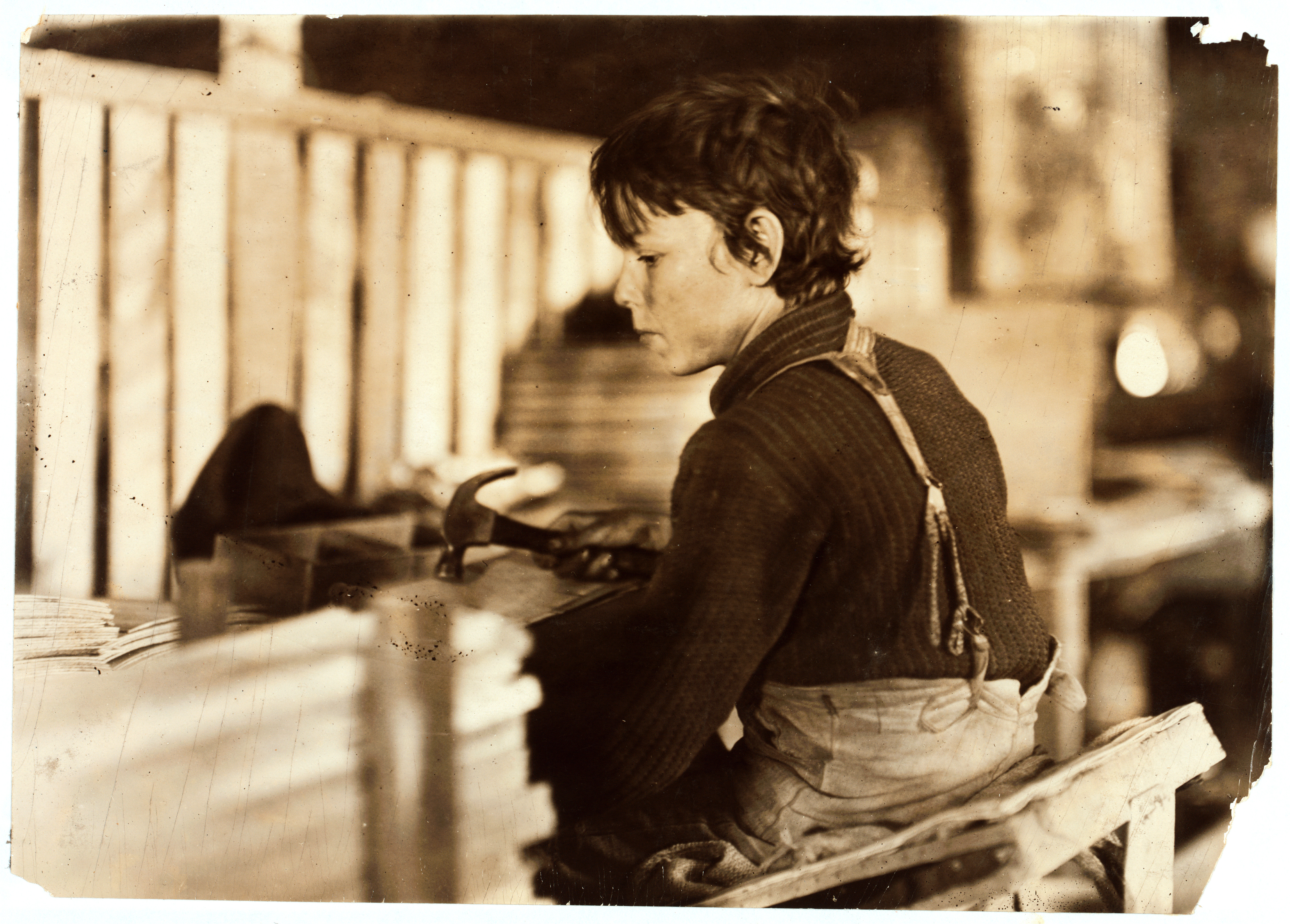This sepia-toned photograph, reminiscent of the 1920s, captures a young boy around 10 years old, deep in concentration as he works with a hammer. The image's palette gives off a vintage feel, blending black, white, and an orange hue. The boy, seated on a tilted bench, has a serious expression and is engrossed in hammering a nail into a piece of wood. He wears a dark-colored striped collared shirt and a pair of light-colored pants held up by suspenders, visible as straps crossing over his back. His hair is disheveled, and there are smudges of dirt on his face, hinting at a long day of labor. Surrounding him, stacks of wood are piled high on the left, and a wooden fence or wall stands in the blurred background. The entire scene is bathed in an atmosphere of hard work and earnest dedication.